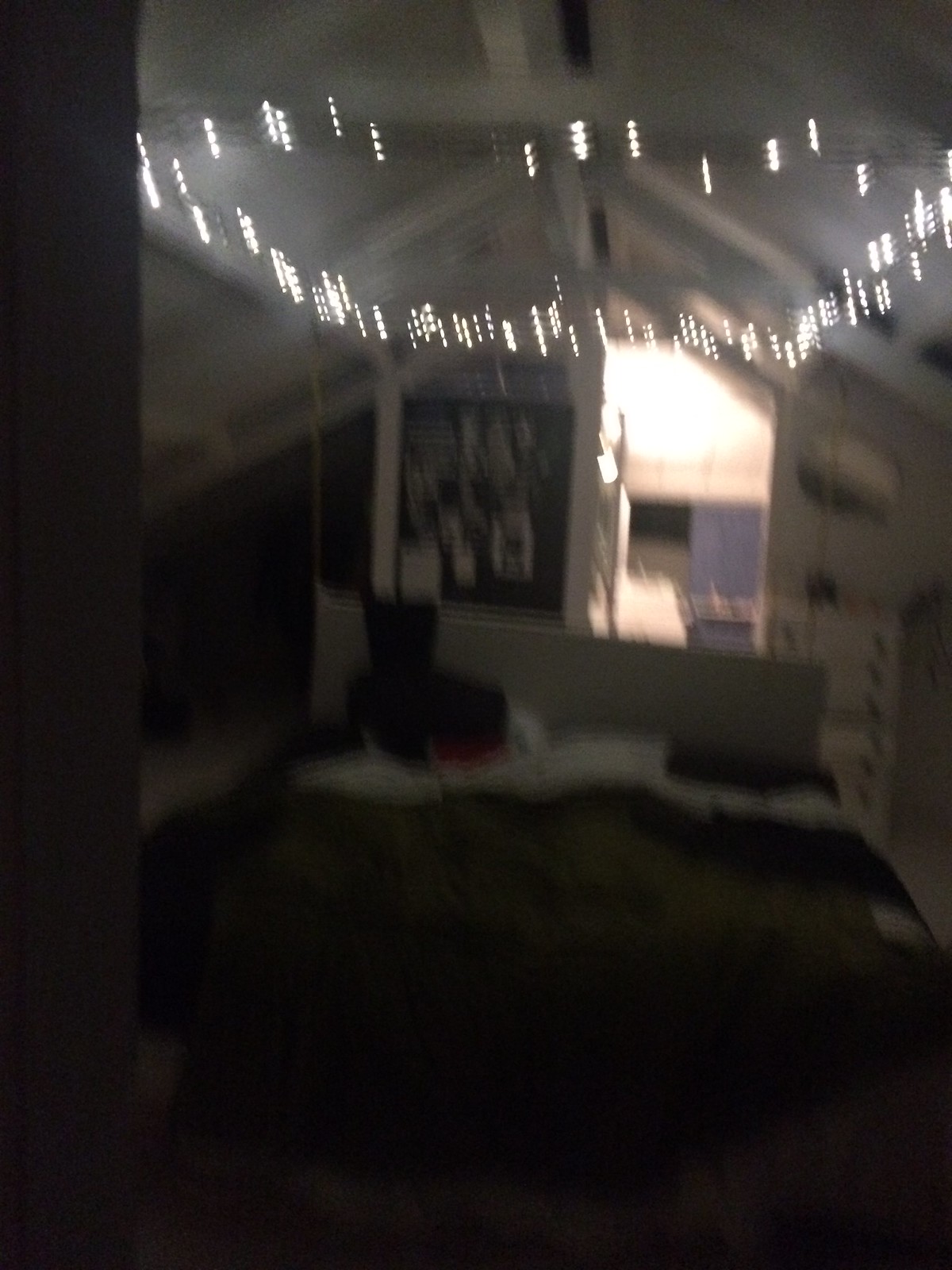The photograph depicts a blurry interior of what appears to be an attic bedroom. The image suggests motion, making the details hazy. At the center is a double bed with mixed bedding—a dark or green quilt, white sheets, and dark pillows. The bed features a white headboard, and behind it is a bulletin board adorned with photos or notes. The room is dimly lit, primarily by white fairy lights arranged in a square above the bed, casting a glow in an otherwise dark space. To the right of the bed stands a white chest of drawers, while on the left side, the ceiling slopes down, enveloping a darkened area. The peaked ceiling, supported by white wooden beams, reinforces the cozy, attic-like atmosphere. An opening behind the bed leads into a lit room with bluish walls, contributing to a slight sense of depth in the photograph.